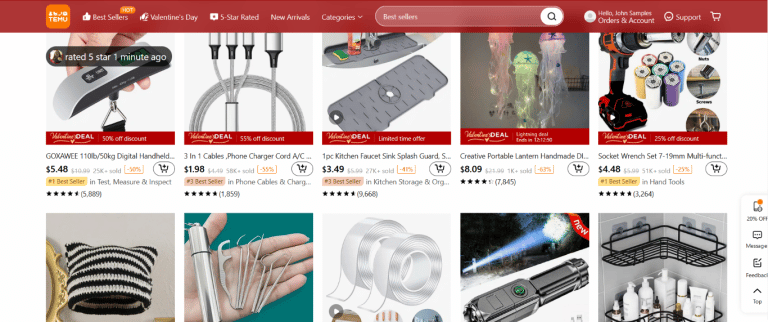The image depicts the landing page of Teemo, a retail website. In the top left corner, the Teemo logo is prominently displayed in orange, marking the brand's identity. To the right, there are navigational options labeled "Best Sellers," "Valentine's Day," "5 Star Rated," "New Arrival," and a dropdown menu for various categories. Adjacent to the categories is a search bar, followed by icons for login, support, and a shopping cart.

Below this header section, the page showcases a series of product images available for purchase. Featured items include a digital handheld scale priced at $5.48, a set of 3-in-1 phone charger cables, an AC unit for $1.98, a one-piece kitchen faucet sink splash guard for $3.49, portable lanterns priced at $8.09, and a socket wrench for $4.48. Additionally, there are images of a hat, toothpicks or floss set, tape, a flashlight, and bathroom shelves; however, their prices are not fully visible or are out of frame.